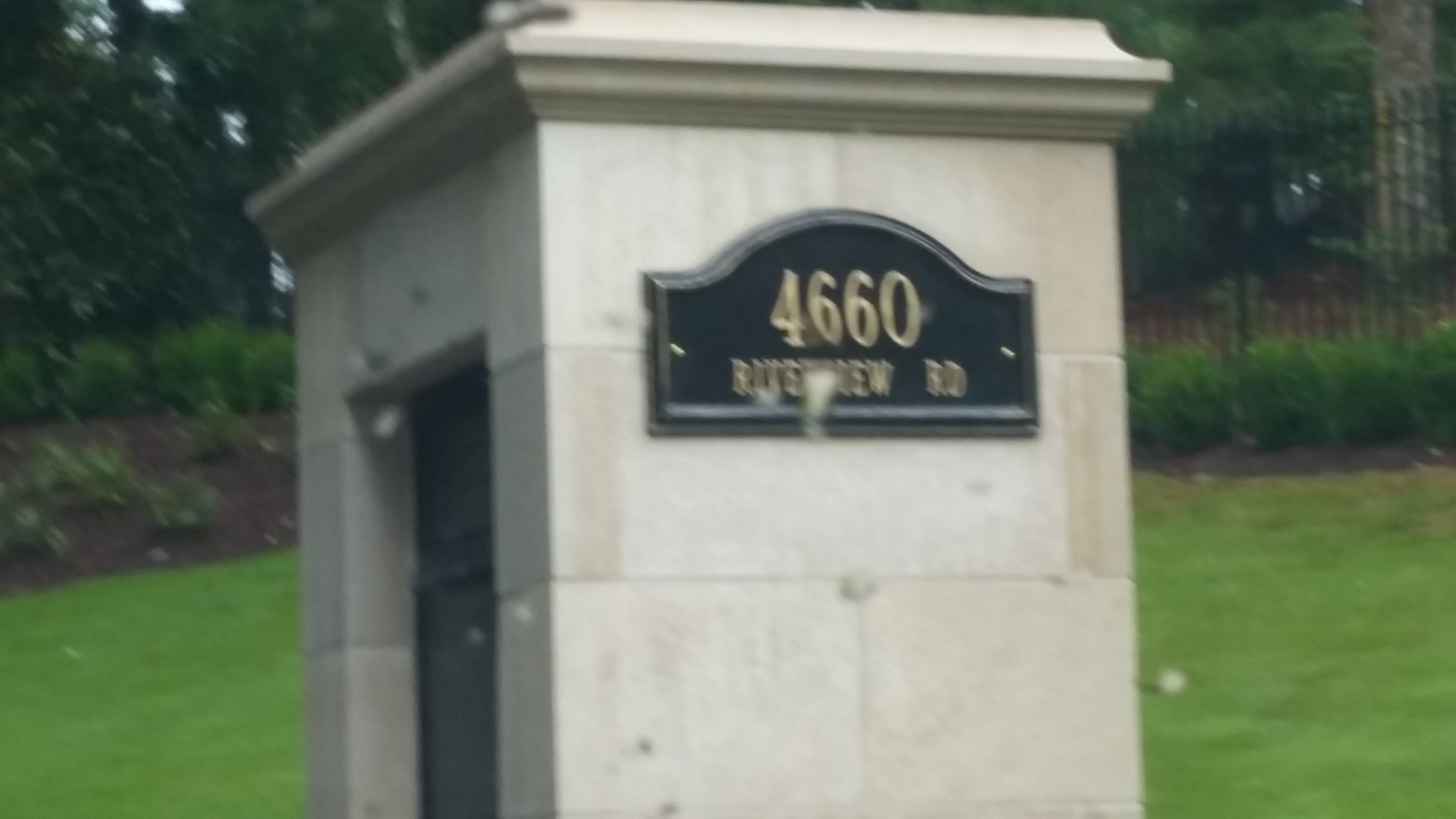A serene green yard is enclosed by a black metal fence. To the left, a modest garden flourishes amidst towering trees, allowing small glimpses of blue sky through their branches. Dominating the scene is a small concrete building with a distinct gray door. Adorning the building is a black sign with the numbers "4660," but only a partial view of the words "Buttersview Road" can be seen. Surrounding the building are large concrete blocks. In the middle of the yard, a small white ball rests, adding a subtle focal point to the tranquil setting.